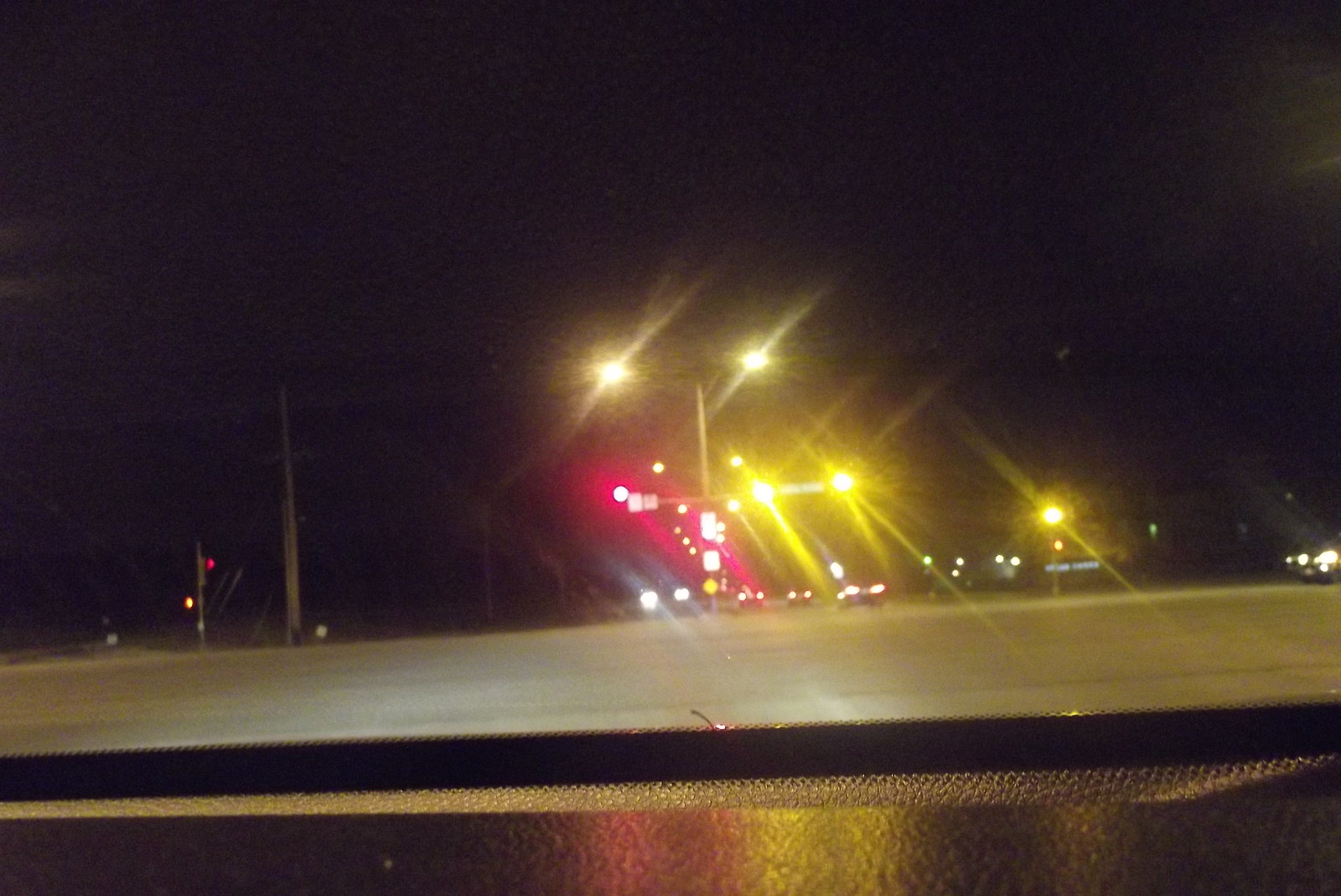In this nighttime outdoor scene, the sky is a deep, impenetrable black, serving as a backdrop for a cluster of streetlights that beam intensely into the darkness. The white streetlights dominate the scene with their glowing intensity, while numerous bright yellow lights add warmth and vibrancy. In the distance, hints of red lights provide additional color depth. The headlights and taillights of cars are visible as they navigate down the streets, casting a dynamic energy into the stillness of the night. Stars manage to peek through the urban glow, adding a touch of celestial beauty to the scene. A traffic light stands prominently, casting its regulated colors onto the road below. The roadway itself features alternating bands of gray and deep black, with stripes crisscrossing in a pattern, where the wider black band contrasts sharply with its thinner counterpart, creating a visually striking composition.